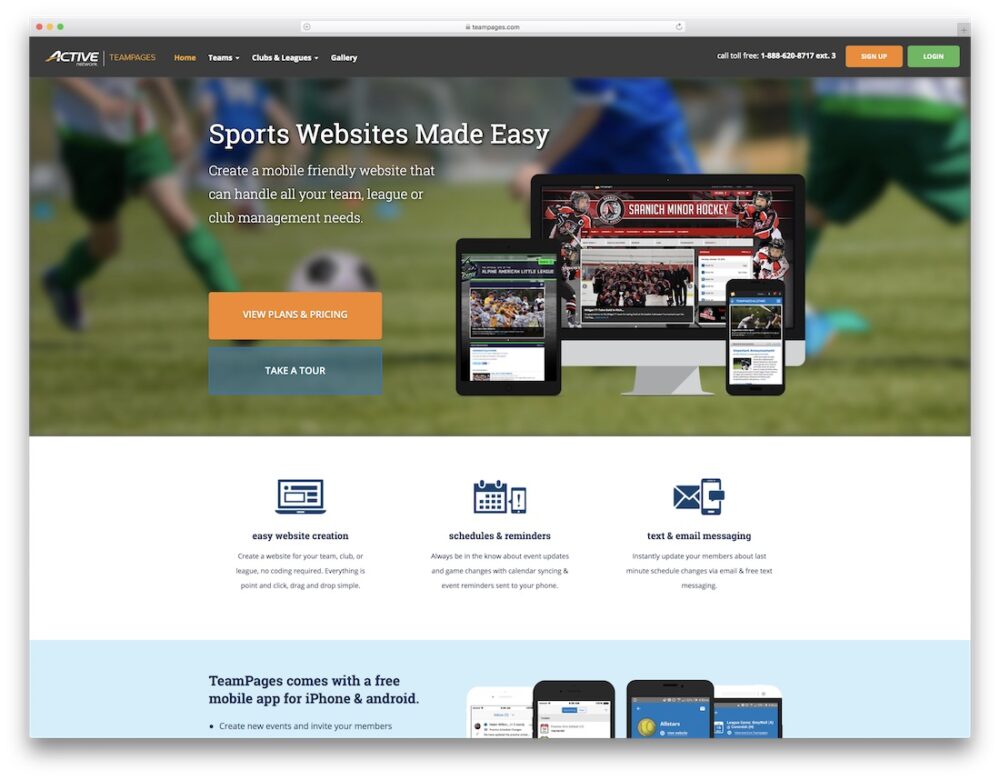This vibrant image, sourced from a sports-oriented website, showcases how effortlessly you can create a mobile-friendly platform for managing your team, league, or club needs, without any coding skills. The website promotes easy website creation with point-and-click, drag-and-drop simplicity. Prominent buttons on the page include an orange "View Plans and Pricing" button and a gray "Take a Tour" button. 

In the background, a dynamic soccer game unfolds on a lush green field. A black and white soccer ball rests on the grass, with a nearby player clad in green shorts and knee pads, ready to make a move. Other players, dressed in either blue or green uniforms, can be seen actively engaging in the match. The functionality of the site ensures that team members stay informed about event updates and game changes through calendar syncing and phone reminders.

Additionally, the image highlights that the Team Pages feature includes a free mobile app available for both iPhone and Android users, blending convenience with real-time sports management.